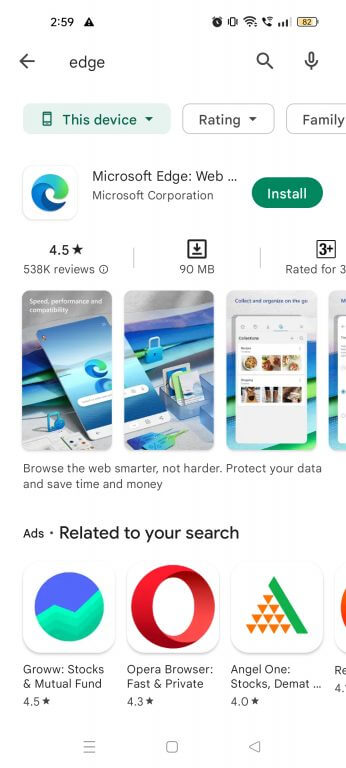This image is a screen capture of a cell phone displaying the App Store page for the Microsoft Edge web browser app. At the top right corner of the screen, the battery icon shows a charge of 82%, followed by three bars indicating cell signal strength. Next to the signal bars are icons representing cellular connectivity, Wi-Fi status with up and down arrows, and a rectangle icon, possibly indicating screen rotation lock. Adjacent to these is an alarm clock icon. On the far left, the time is displayed as 2:59, along with a triangle containing an exclamation point, potentially indicating a notification.

Below this status bar, the display shows black text reading "Edge" accompanied by a left-pointing arrow. To the right of this arrow, there is a magnifying glass icon representing search functionality, followed by a microphone icon suggesting voice input capability. 

Below these icons, three labeled boxes appear: the first one reads "This Device," indicating the app's installation destination, the second one reads "Rating," and the third says "Family," likely categorizing the app's content.

Further down the screen, the familiar Microsoft Edge icon, which is a blue and green swirl, is prominently displayed. Next to the icon, the text reads "Microsoft Edge: web…" followed by "Microsoft Corporation." To the right of this text, a prominent green button labeled "Install" is visible.

Additional information provided includes the app's rating of 4.5 stars out of 5, based on 538K reviews, the app's size of 90MB, and an age rating of 3+, indicating it is suitable for ages three and up.